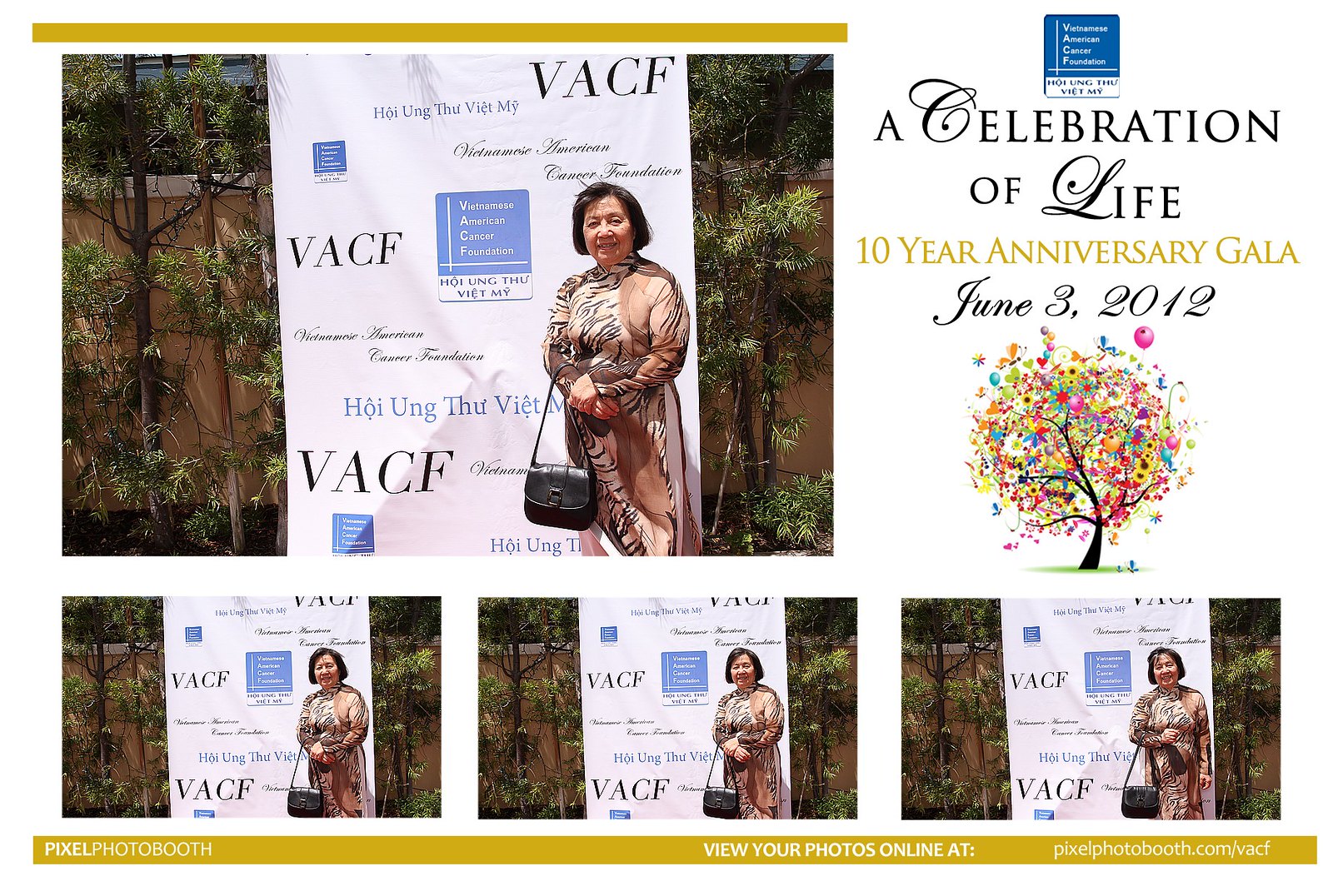The image resembles a postcard and features a collage of photos from an event celebrating the Vietnamese American Cancer Foundation (VACF). The central and largest photo, positioned in the upper left, depicts an older Asian woman with short, dark hair and a black purse on her right forearm. She is wearing a beige dress with a tiger-print pattern, standing in front of a white banner that displays the VACF logo. The logo itself, found in the top right, is a blue and white square resembling a book, with the foundation's name written in both English and Vietnamese.

The background shows plants and a beige wall, indicating an outdoor setting under bright daylight. Adjacent to the banner, there's the phrase "A Celebration of Life, 10-Year Anniversary Gala, June 3rd, 2012" written in stylish fonts. Below this phrase is a vibrant illustration of a tree with black branches and multicolored leaves, balloons, hearts, stars, and flowers set against a green grass floor.

Beneath the primary photo, there are three smaller, identical pictures of the same woman in slightly different poses. The image has greenish-yellow borders at the top and bottom, with footnotes in the lower border. The footnotes include the text "Pixel Photo Booth," instructions to view photos online, and the website address pixelphotobooth.com/vacf. The overall composition highlights the theme of life celebration and community support, consistent with the mission of the Vietnamese American Cancer Foundation.